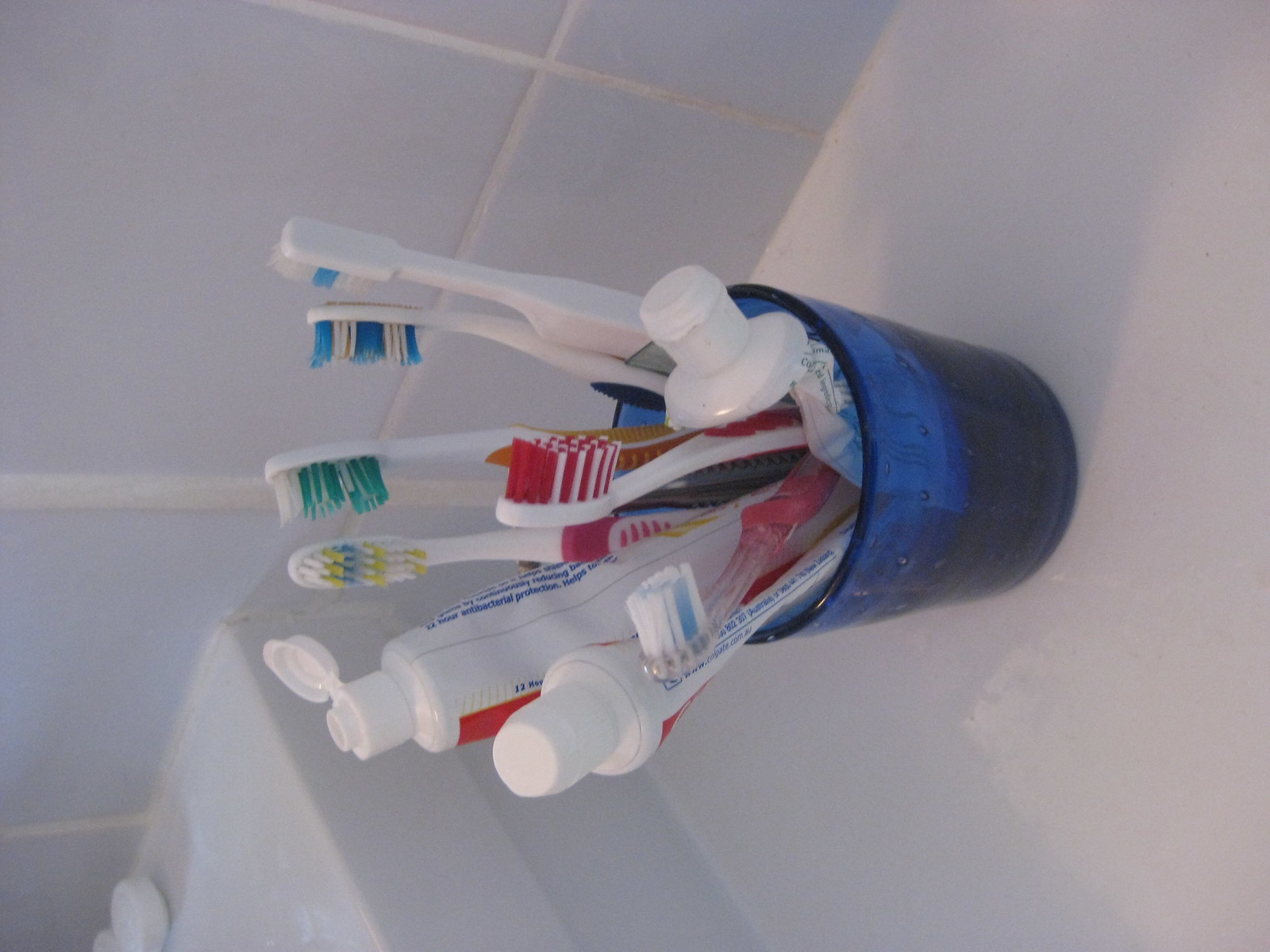The photograph captures a bathroom scene with a focus on a blue cup, which is positioned on a white porcelain sink. The image is taken from a left-side angle, causing the cup and its contents to appear horizontal. The backdrop features light blue or white shiny tiles with white grout. Inside the translucent royal blue cup are six toothbrushes with various colored handles—reds, greens, yellows, blues, and whites. The bristles are predominantly white with stripes of blue and green. Additionally, three toothpaste tubes are also in the cup: one small tube and two taller ones. The cap of the fullest tube is open, and another tube is noticeably more used and wrinkled. The overall bathroom setup includes a reflective white countertop and a barely visible white contact case on the right.